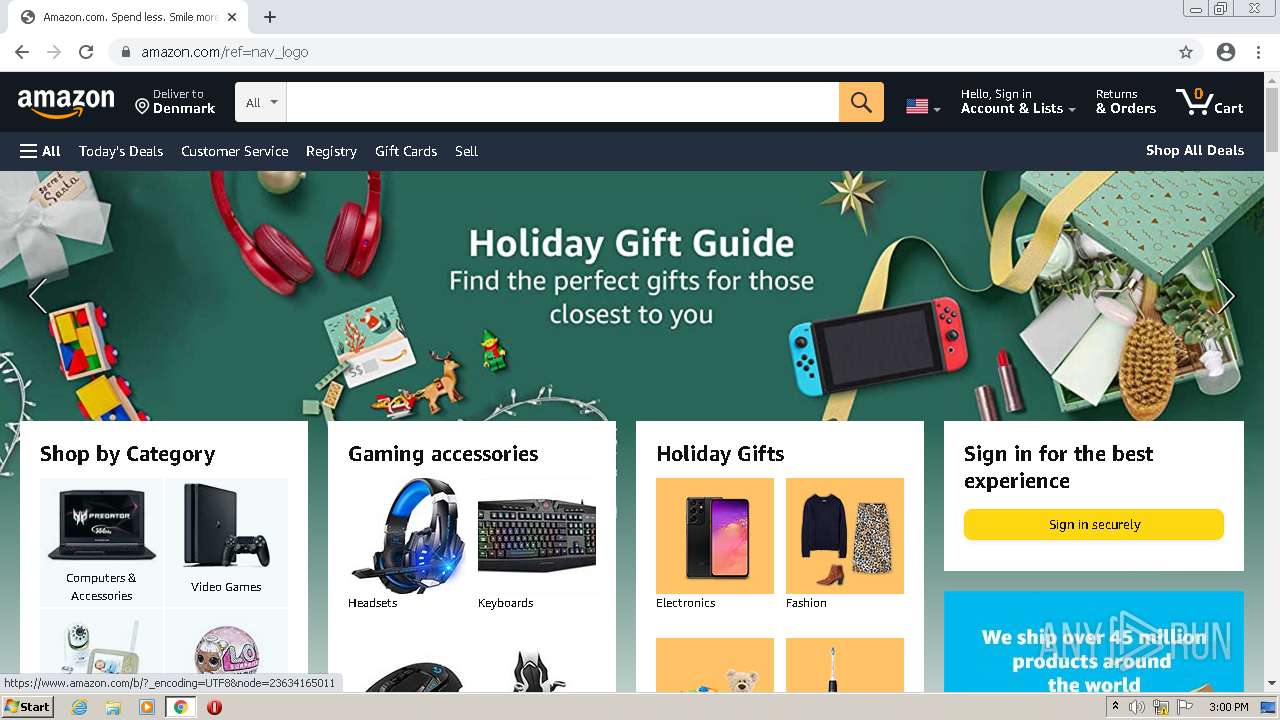This horizontal screenshot captures the Amazon.com homepage, showcasing the website's interface with the address bar prominently displaying the URL. A light gray strip at the very top indicates that this is the only open tab. The Amazon logo on the left, featuring white text and a light yellow arrow, is clearly visible. The setting is localized to Denmark, as indicated by the "Deliver to Denmark" text near the logo.

The main section of the page features a green background with a prominent white text header reading "Holiday Gift Guide: Find the perfect gifts for those closest to you." The products displayed include a pair of red earphones or headphones, a block train set, a Nintendo Switch, a tube of lipstick, and a gift box containing various toiletry items.

Below this section are five clickable categories, four of which are white while the fifth is blue. The categories are: "Shop by Category," "Gaming Accessories," "Holiday Gifts," and "Sign in for the best experience" with a yellow "Sign in securely" button. The blue box beneath these categories states, "We ship over 45 million products around the world."

At the bottom of the image, the user's computer taskbar is visible, displaying the start icon and several other icons, with the system clock indicating the current time as 3:00 PM.